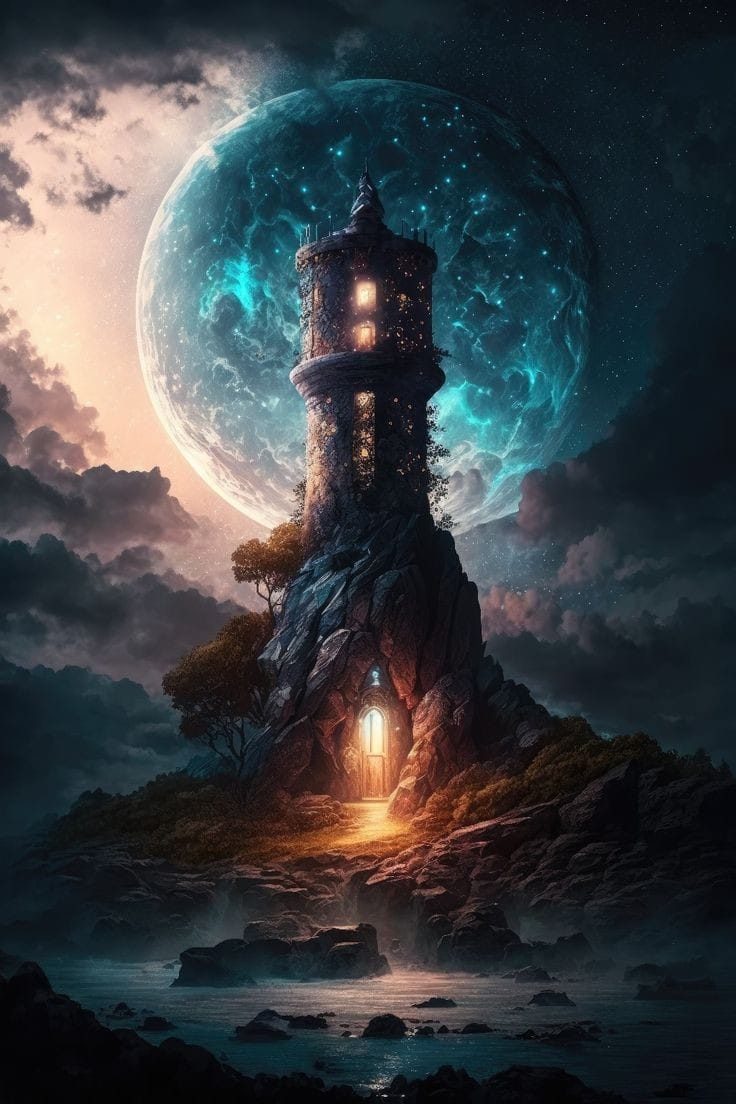This image portrays a fantastical, computer-generated scene set in an otherworldly night. Dominating the center is a tall, slender tower resembling a lighthouse, arising from a narrow, rocky mountain base. The base features a prominently lit entrance set into a cave-like structure. Midway up the tower, trees cling to its left side, adding an element of natural beauty. At the top of the tower, softly glowing windows offer a warm contrast to the darker surroundings. The background is dominated by a large, blue-glowing planet emitting light from various cracks and points, creating an ethereal atmosphere. Surrounding the tower, the sky transitions from a star-studded dark blue on the right to patches of bright light on the left, interspersed with clouds in shades of black, white, and various purples. The overall scene captures the mystical feel of a fantasy landscape, blending earthly elements with cosmic wonder.